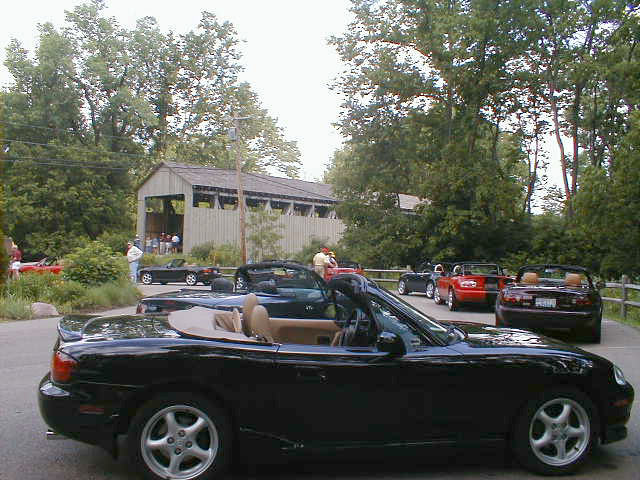The photo captures a daytime outdoor scene at a roundabout-shaped parking area filled with convertible sports cars, reminiscent of a Mazda Miata meet-up. The main focus is a side view of a black convertible with tan interiors and brushed silver rims, its top down and facing slightly sideways. Surrounding it are several more unattended convertibles, including black, red, maroon, and green ones, all parked in varying orientations. In the background, a picturesque covered bridge, painted dark green with barn-like sides, spans over a river and stands among the surrounding trees. People can be seen standing near the left-side opening of the bridge, adding a human element to the tranquil setting.